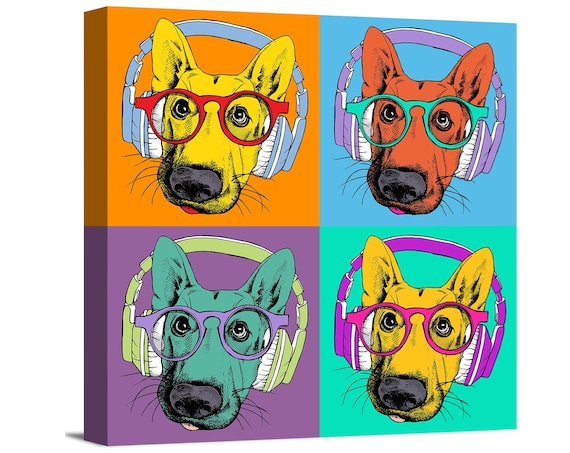This vibrant artwork is divided into four distinct squares, each depicting a stylized dog's head, possibly a Doberman or Greyhound, with sleek fur. The dogs are drawn in varying colors against contrasting backgrounds, each adorned with a unique set of glasses and over-ear headphones. 

In the top left square, a yellow dog with red sunglasses and grey headphones stands against an orange background. The adjacent top right square features an orange dog wearing teal glasses and purple headphones over a blue background. The bottom left square displays a teal dog, accented with purple glasses and green headphones, set against a purple background. Finally, the bottom right square showcases a mustard yellow dog with magenta glasses and purple headphones against a teal background. Each dog's expressive image is further enhanced by their own black noses, adding a touch of uniformity to the diverse and colorful presentation.